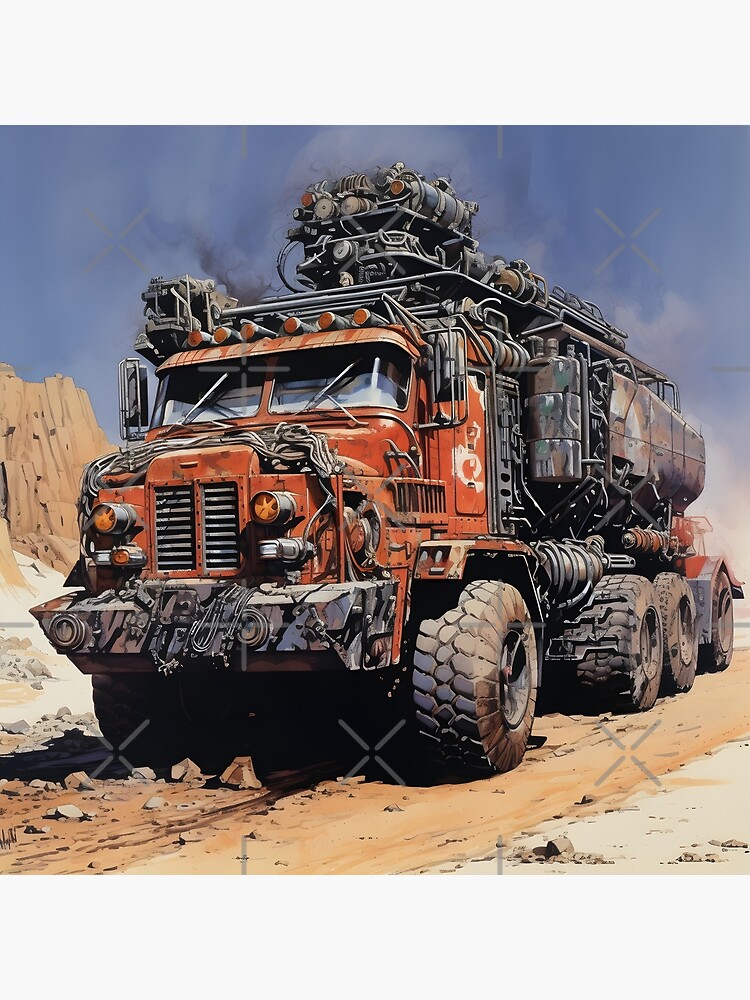In a vivid, comic-style illustration, a massive, worn-down, rusty red truck commands the scene, reminiscent of a Mad Max military vehicle, rumbling down an utterly barren, desert-like dirt road. The landscape features rugged cliff faces to the left under an expansive blue sky, devoid of clouds, enhancing the stark isolation of the setting. The truck is depicted with enormous, off-road wheels, showing four from an angled side view, which underscore its formidable size. Its metallic storage tank at the back, likely intended for some heavy-duty purpose, integrates with an elaborate array of grey canisters and piping on top, suggesting a complex fueling system. This vehicle, emitting various types of smoke and steam, brims with an assortment of hardware, blending an imaginative jumble of elements that evoke a dystopian utility. The entire scene is marked with subtle watermarks, adding a layer of artifice to this intriguingly detailed creation.